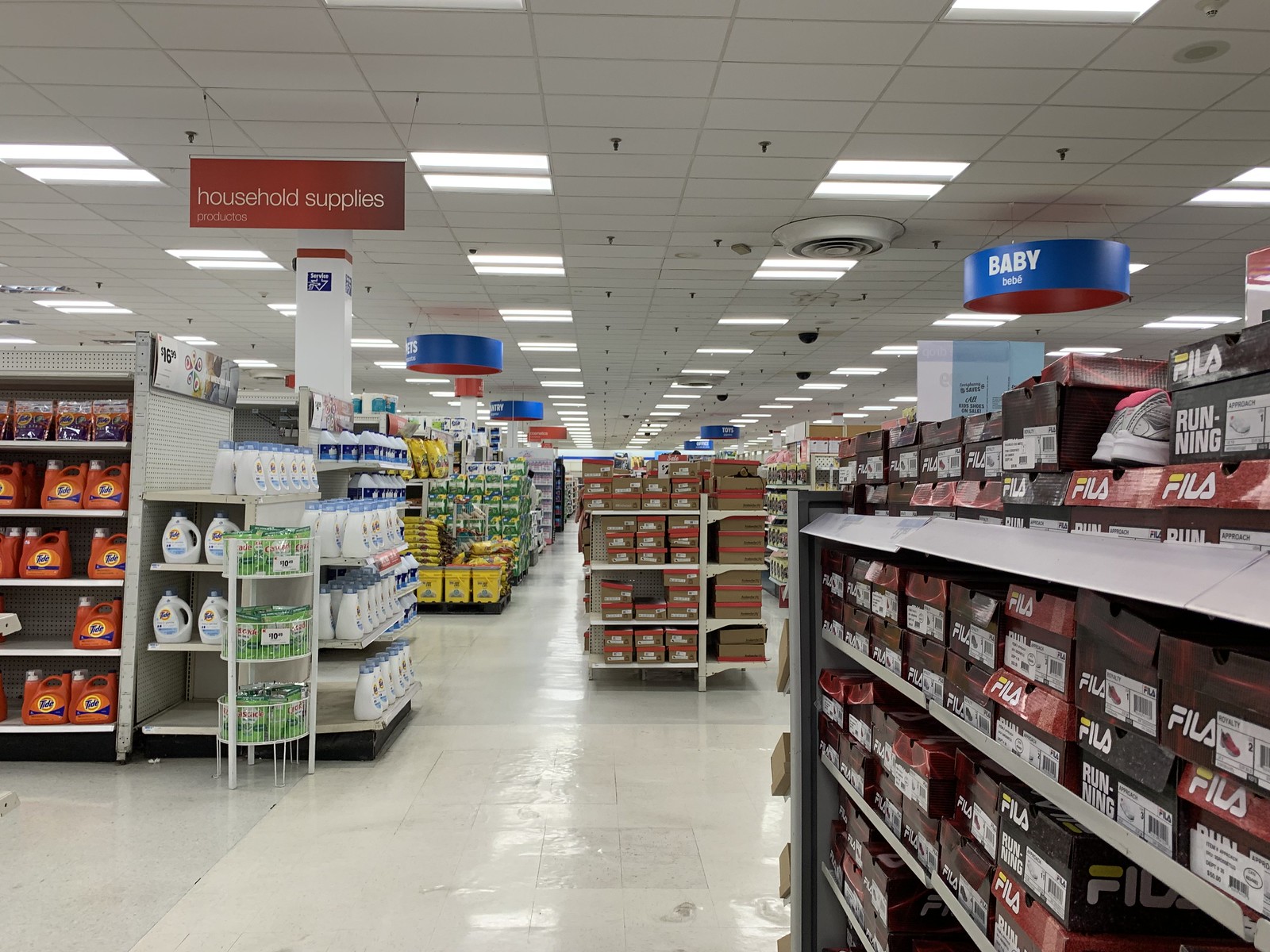The image captures a detailed interior view of a well-worn big box variety store, brimming with a diverse range of products. The aisle in focus features a display of shoes and boots, while a prominent sign indicates sections for household supplies and baby items. Large jugs of clothes washing detergent line the left side of the aisle, with an end-of-aisle display showcasing "free and clear" detergent in recognizable white bottles with blue tops. In the background, shelves stocked with bags of birdseed and charcoal are visible, along with running shoes and beautifully designed boxes. Several pairs of shoes are nestled between these boxes, adding to the eclectic mix. The ceiling is equipped with monitoring cameras, a sprinkler system, vents, and acoustical tiles, all bearing smudges and marks that hint at the store's age. The tiled floor, showing signs of heavy use and cart traffic, further emphasizes that this store has been a long-standing fixture, characterized by its extensive and varied inventory.